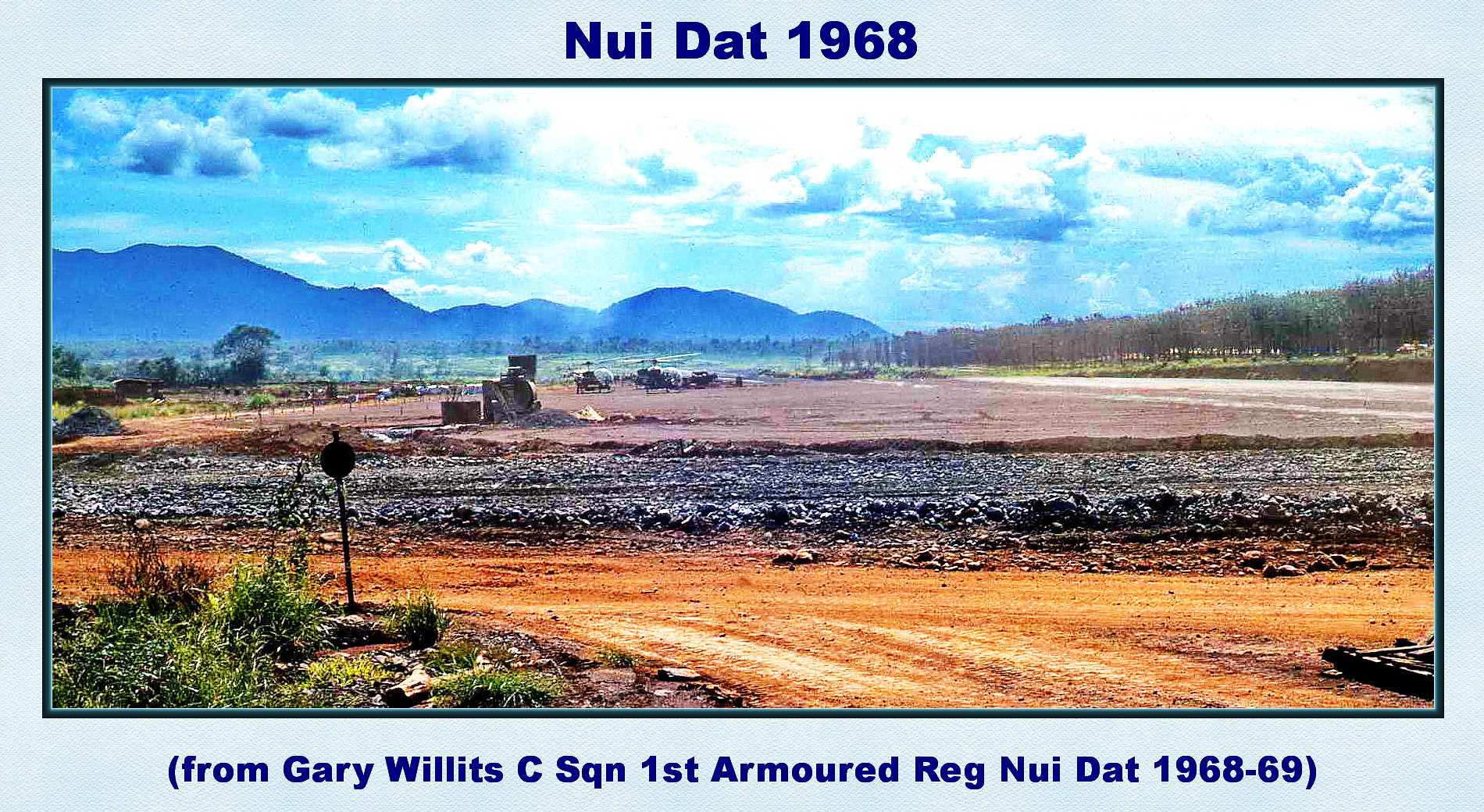This landscape image, titled "Nui Dat, 1968," originates from Vietnam and was captured by Gary Willits of the First Armored Regiment during 1968-69. The photograph is bordered by a light blue frame with dark blue text above and below it. The title at the top reads "Nui Dat, 1968," while the caption below attributes the image to Gary Willits, detailing his regiment. The scene within the image is characterized by a vast, largely barren field with a muddy foreground and a dirt road featuring a small sign, possibly a stop sign, veering out of view. The center of the image shows disturbed black and brown dirt, suggestive of recent activity, possibly by machinery distantly visible. The landscape includes a strip of green grass adjacent to the road and a dense line of trees to the right. The horizon is dominated by a dark, gray-blue mountain range extending from the left and leveling out towards the right, under a sky filled with dramatic white clouds partially obscuring the sun. The photograph is emblematic of the realism style, blending photographic elements with representational details to vividly capture a moment in Nui Dat’s history.